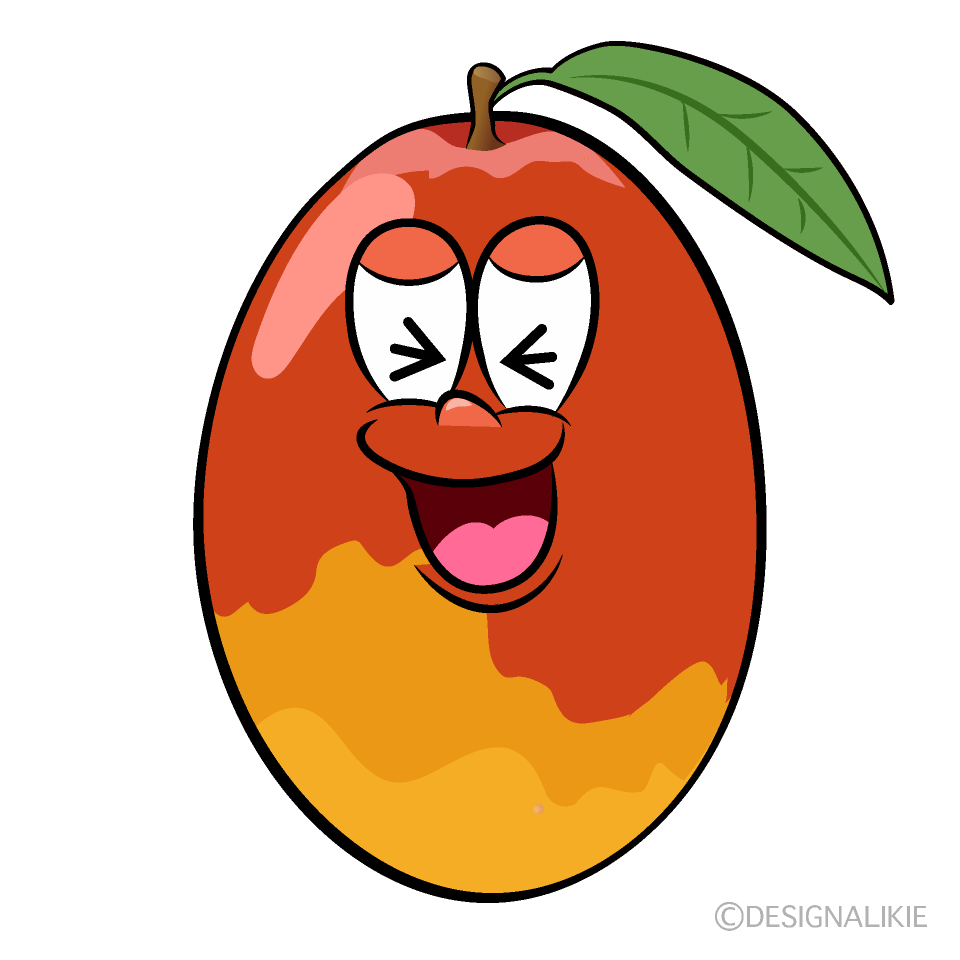The image depicts a cartoon-like character with an oblong shape, reminiscent of an apple. Topped with a brown stem and a single green leaf branching to the right, the character stands out with a vibrant red upper section accented by white splotches that suggest reflections. The middle section transitions into an orange hue forming a C-shape, while the base is a blend of darker gold tones. 

The character’s face is expressive: it squints with eyes that are shaped like black arrows pointing in opposite directions - right and left. It also has large, oval eyes with three small lines inside, complemented by pinkish eyelids. The nose is a gradient of colors – predominantly pink in the center with orange on the upper part and red on the lower part. Its mouth is outlined in black, displaying a maroon interior and a pink tongue, giving the impression of laughter. This whimsical, ovate figure is set against a plain white background, possibly hinting at a designer’s logo or a playful illustration.